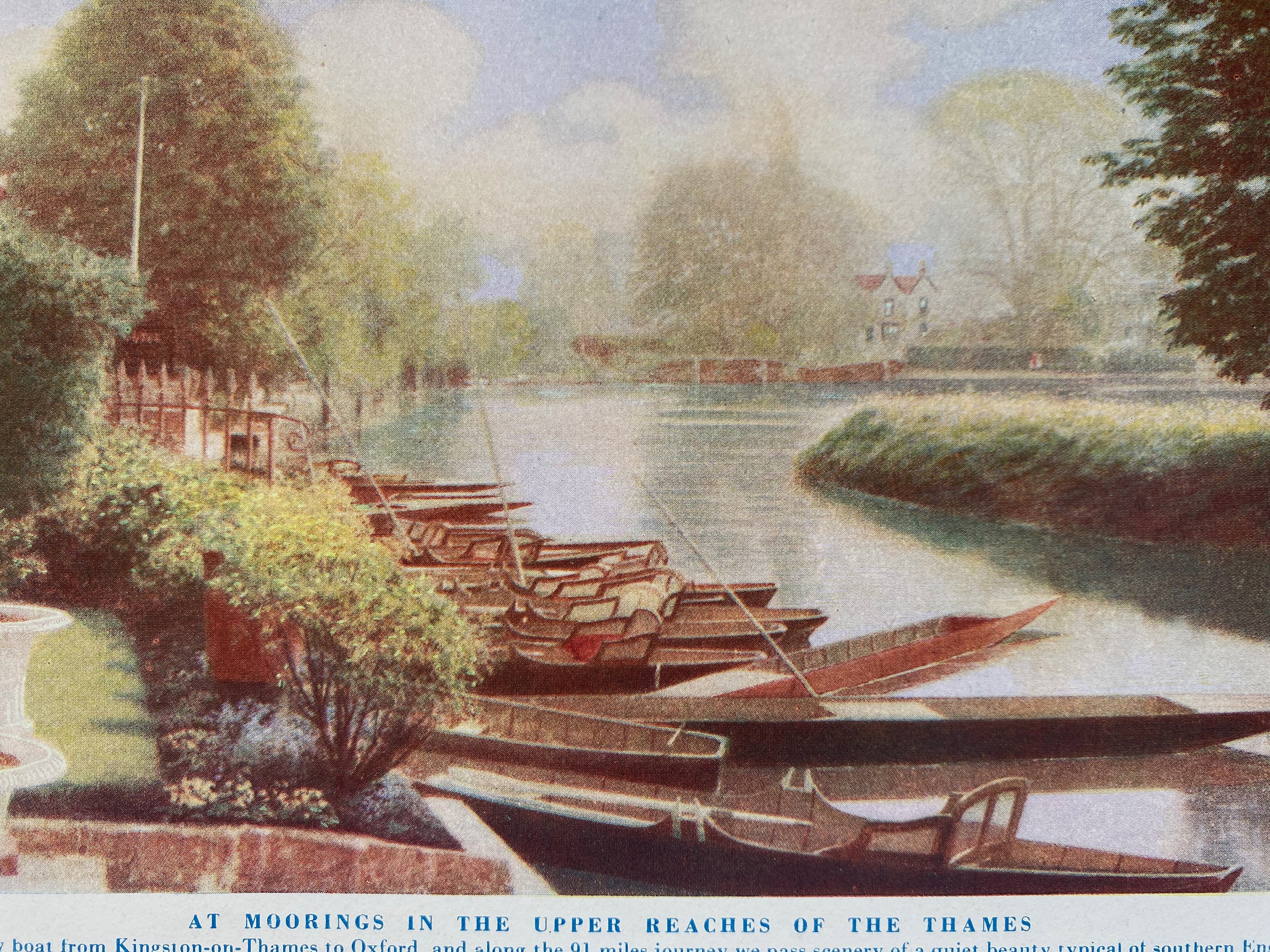This is an old-fashioned painting titled "At Moorings in the Upper Reaches of the Thames," indicated by blue letters on a gray box at the bottom of the image. The painting features a tranquil riverside scene, emphasizing a series of dark brown wooden boats, or canoes, tightly lined up along a riverbank in the foreground. To the left of the boats, there's a concrete embankment adorned with well-manicured shrubs and trees, and two tall white planters in the far right corner. The river wraps around a little grassy island in the center-right, which hosts a large tree. Across the water on the right side, a brown house with a red roof and gray sides peeks through the dense foliage, accompanied by a mix of large trees and smaller green bushes lining the shoreline. In the background, the river continues to wind through a landscape of serene greenery under a light blue sky dotted with white clouds. The overall color palette of the painting is somewhat worn and drab, adding to the historical feel of the scene. The image captures a peaceful, rustic riverside vista enriched with natural and architectural details.